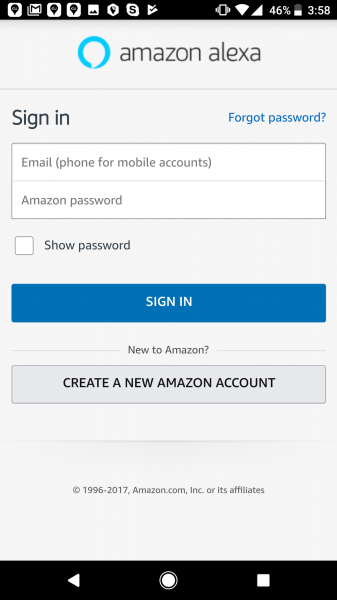The screenshot depicts a vertical capture from an Android mobile phone at 3:58 PM with a 46% battery level. The screen displays the login page of the Amazon Alexa app. At the top of the screen, various notifications are visible, including ones from Skype, Gmail, and an unidentified app, as well as a phone call notification.

The main content of the screenshot shows the Amazon Alexa login interface, featuring the Amazon Alexa logo prominently at the top. Below the logo, there are input fields for 'Email or mobile phone number' and 'Amazon password,' accompanied by a 'Show password' checkbox. A large blue 'Sign-In' button is located immediately below the password field. Beneath this, there is a prompt that reads "New to Amazon?" followed by a grey button labeled 'Create a new Amazon account.' The page also includes a 'Forgot password?' link in blue text. At the bottom, the screen displays a footer with text indicating "© 1996-2017, Amazon.com, Inc. or its affiliates."